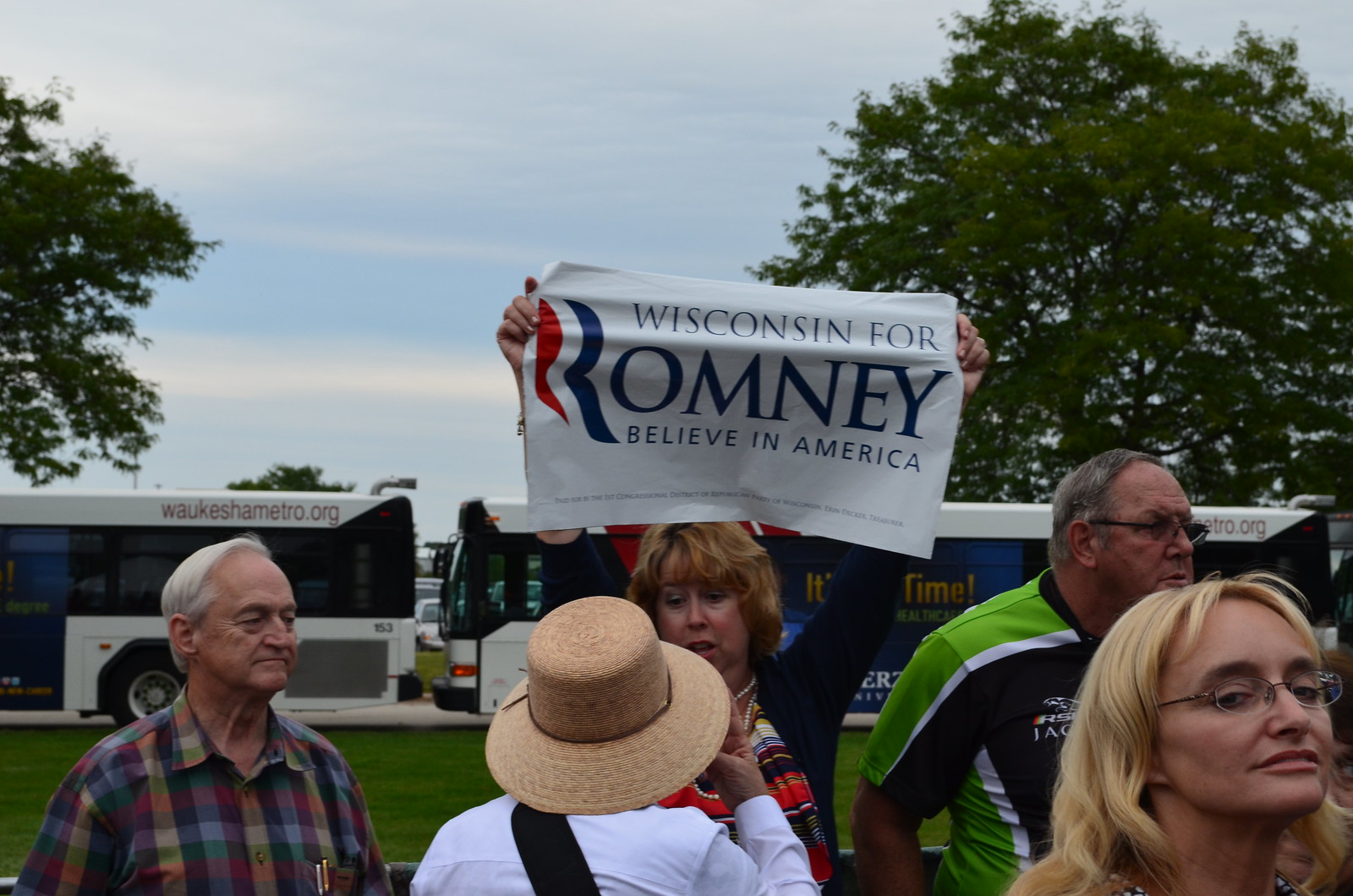An outdoor photograph captures a group of five white individuals, consisting of three women and two men, ranging from middle-aged to elderly, dressed in colorful leisure clothing. Prominently, a late middle-aged woman stands in the center, holding aloft a slightly wrinkled white banner with blue text and a red, white, and blue "R" that reads, "Wisconsin for Romney, Believe in America." The group poses on a green turf with a backdrop of two or three buses on a road, one marked with "WaukeshaMetro.org" and another possibly displaying a Romney sign. Further back, a few large green trees frame the scene against a mostly pale blue sky streaked with white clouds, suggesting an overcast, yet somewhat clear day, likely around midday. This setting is indicative of a political rally for Mitt Romney.